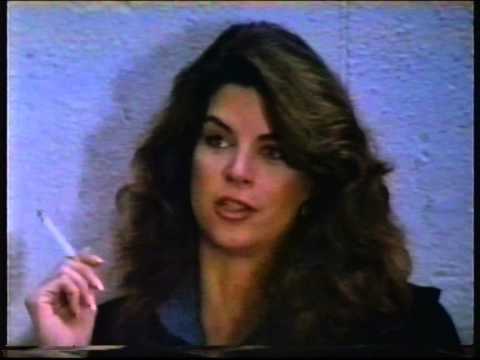In this image, Kirstie Alley is featured in a close-up shot that appears to be taken from a recording, most likely from a VHS tape, given the noticeable distortion at the top and bottom of the frame typical of overplayed tapes. She stands against a blue, slightly periwinkle cinder block wall, looking directly into the camera with her mouth open as if caught mid-conversation. Her thick, dark brown hair, parted on the side, cascades in waves to her shoulders. She wears a dark jacket or sweater over a lighter blue shirt, with a faint trace of reddish lipstick accentuating her animated facial expression. In her right hand, adorned with white nail polish, she holds a long white cigarette. Her eyebrows are neatly plucked and arched, framing her expressive eyes. This snapshot distinctly captures her stylish and animated presence.